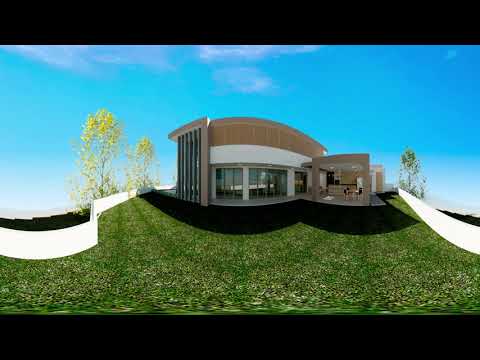The image is a 3D rendering of a luxurious, modern house presented from a panoramic, 360-degree perspective, showcasing the backyard. The house exhibits unique architecture, featuring a curved front with tall windows spanning two or three stories. It includes an outdoor cooking area with a counter, fridge, and a table surrounded by chairs, perfect for dining and conversation. On the right side of the image, there's a long table and a shorter table with three chairs. To the left of the building, a white fence borders lush green grass and a couple of light green trees, with one tree positioned to the right. The house's exterior includes three white-painted pillars and an inverted L-shaped structure with a wooden finish at the top. There is a pathway leading from the house, extending downhill on the right side. The shadows of the house are clearly defined on the grass. The background features a blue sky with partial white clouds, adding to the crisp and detailed quality of the rendering, which includes a black border at the top and bottom of the image.